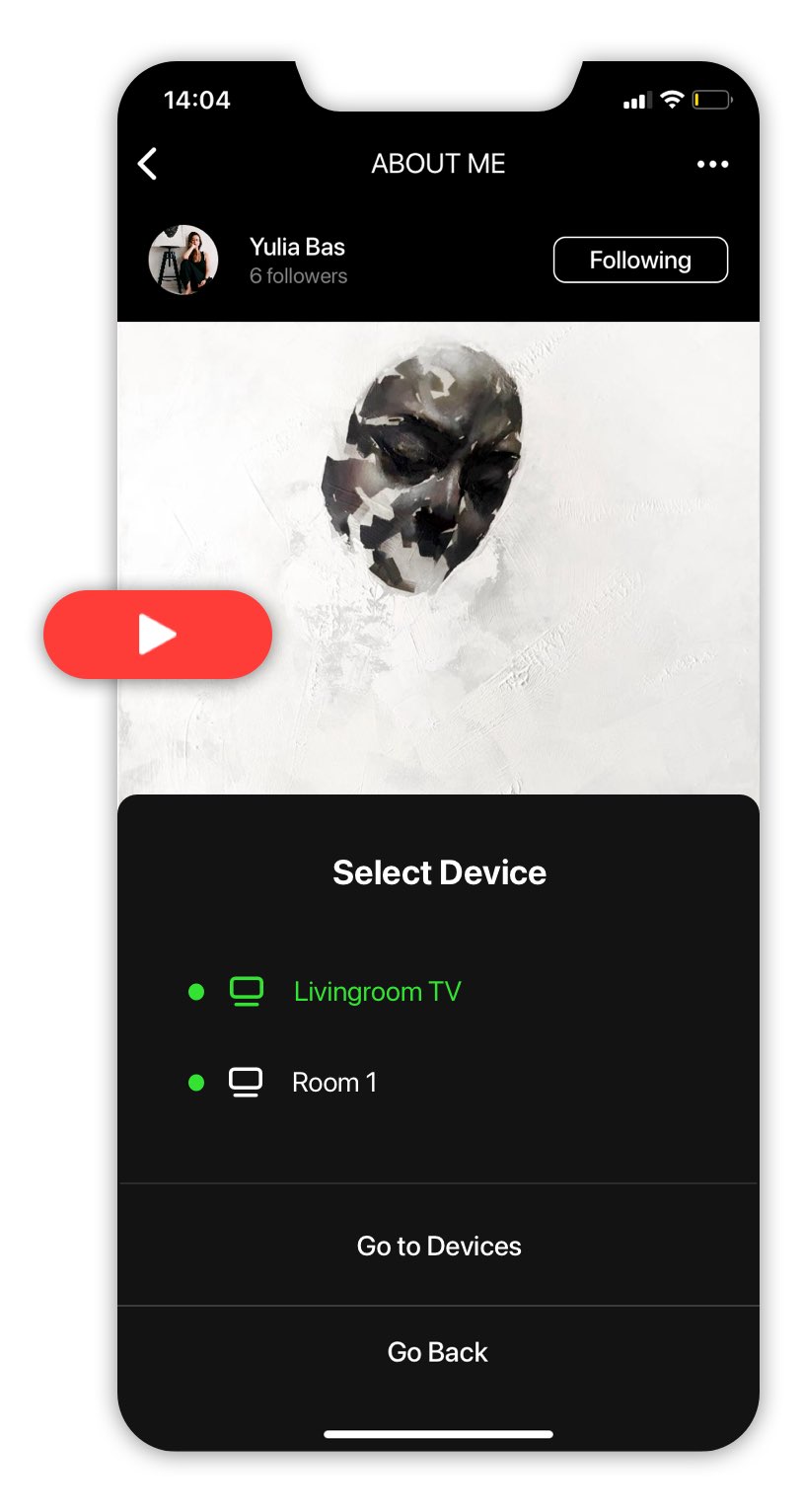This detailed caption provides a comprehensive description of the smartphone mock-up screenshot you provided:

"Presented is a mock-up screenshot of a modern smartphone interface, prominently featuring no chrome but the outline of the device's screen with elegantly curved edges. A subtle chin at the top is visible, framing the display which is enveloped by a pronounced drop shadow along the top, sides, and bottom, against a crisp white background.

The upper section of the screen showcases a black bar displaying the time in a digital font reading '14:04'. To the right of this, perched on the left side of the chin, there are three signal bars, a full Wi-Fi signal, and a battery icon indicating approximately 10% charge.

Beneath this status bar, the interface includes a 'Back' arrow on the far left, an 'About Me' section centered, and three vertical dots on the right edge, indicating more options. This profile belongs to 'Yulia Bass,' with a vibrant color photograph depicting a woman dressed in a black tank top and possibly black jeans, sitting against a white wall. Beside her is an old-fashioned stool with a circular, threaded top, on which a piece of art sits. Her pose is thoughtful, with one hand resting on her knee and the other under her chin.

A button next to her name signifies the user is following her. Below this section, an artist's abstract drawing of a face is highlighted, featuring intriguing, floaty elements. Overlaying the left side of this artwork is a prominent, red YouTube-like play button with a white triangle in the center, appearing to float outside the phone's frame.

Further down the interface, the option to 'Select Device' for streaming is presented with two choices: 'Living Room TV' and 'Room 1', with the former highlighted in green, indicating it is currently selected. At the very bottom, dark gray buttons offer options to 'Go to Devices' or 'Go Back,' completing the lower portion of the screen."

This description encapsulates the layout and elements visible in the screenshot in a structured and detailed manner.